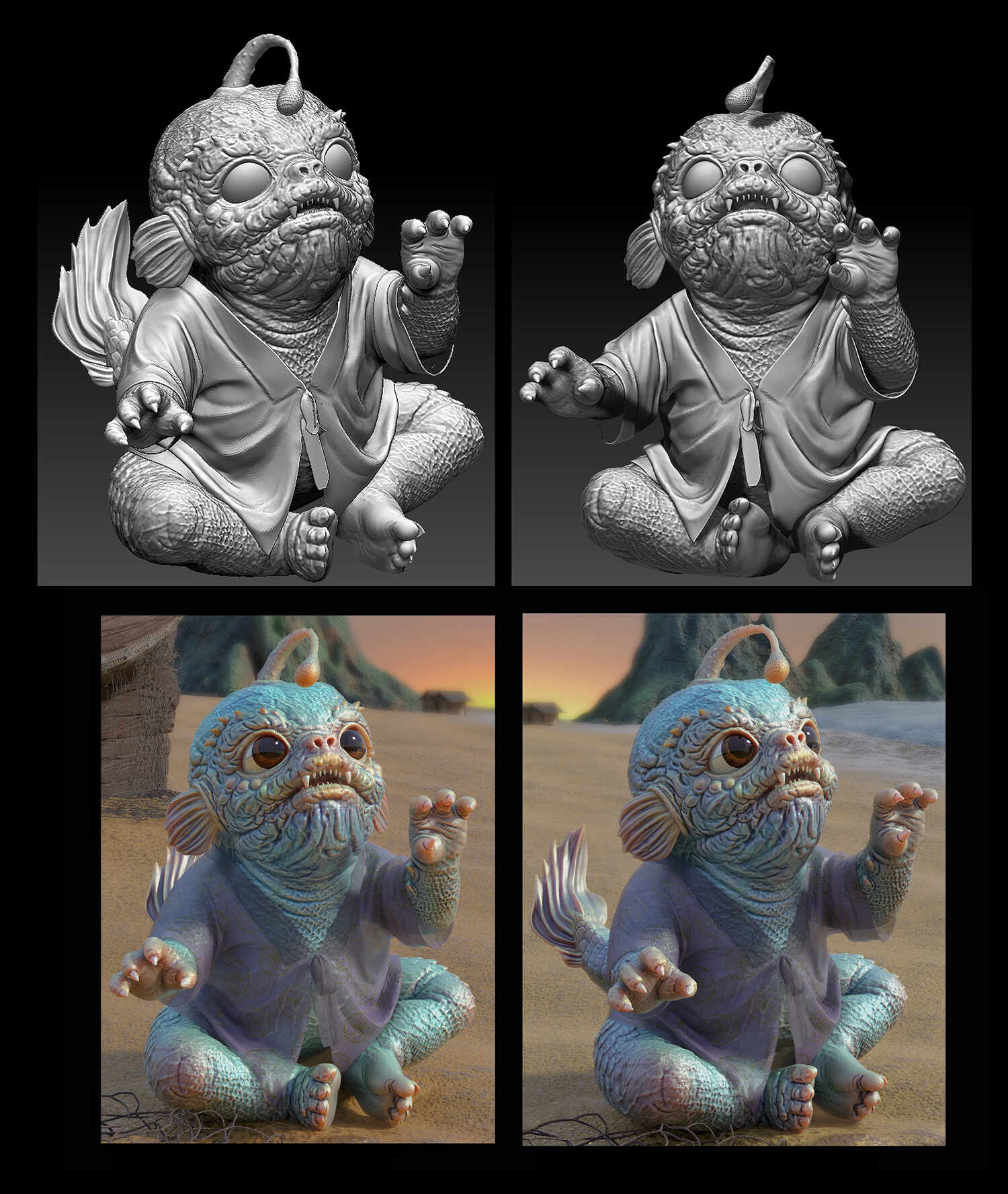The image showcases a 3D character design that transitions from an unrendered CAD model to fully rendered illustrations, incorporating elements of both sci-fi and fantasy. This small alien baby, bathed in shades of blue with scaly skin and flesh-toned fingers, features distinct characteristics such as an antenna reminiscent of an anglerfish's lure, fin-like ears, and a tail suggesting a lineage akin to fish or dragons. The CAD model, in monochrome grays, highlights its detailed, scalable anatomy, while the rendered images bring it to life with vibrant hues. The character is adorned in a purple tie-together vest, standing out against its blue body. It has large, soft brown eyes that evoke a sense of innocence and curiosity, consistent with its baby-like nature. Posed sitting on what appears to be an alien beach with mountains and water in the backdrop, the creature gazes out inquisitively, as if captivated by something unseen, like a butterfly, adding to its endearing and exploratory demeanor.